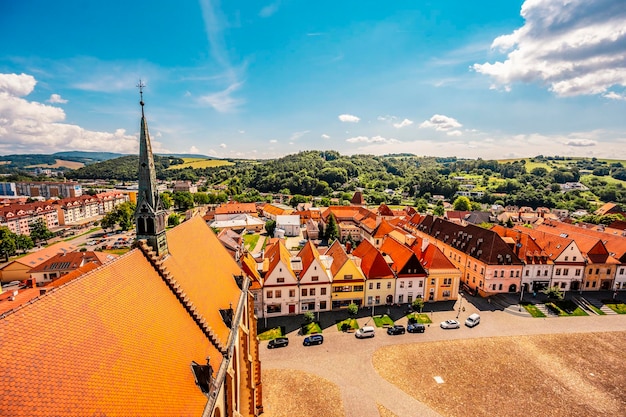This drone shot captures a vibrant European village nestled in the countryside. The closest and most prominent building is a church with a steep, high-peaked orange-red roof featuring stairs that lead up to its bell and steeple. The closely packed two-story homes, uniform in their interconnectedness and warm orange-red roofs, create a dense, cohesive appearance as they line the narrow streets. Cars are parked out front of these homes, indicative of a small but active community. In the background, a hilly landscape filled with lush green trees stretches out, suggesting a rural setting that blends seamlessly with the village. The scene is bathed in bright daylight under a vivid blue sky adorned with fluffy white clouds, enhancing the picturesque and serene atmosphere of this quaint European village.